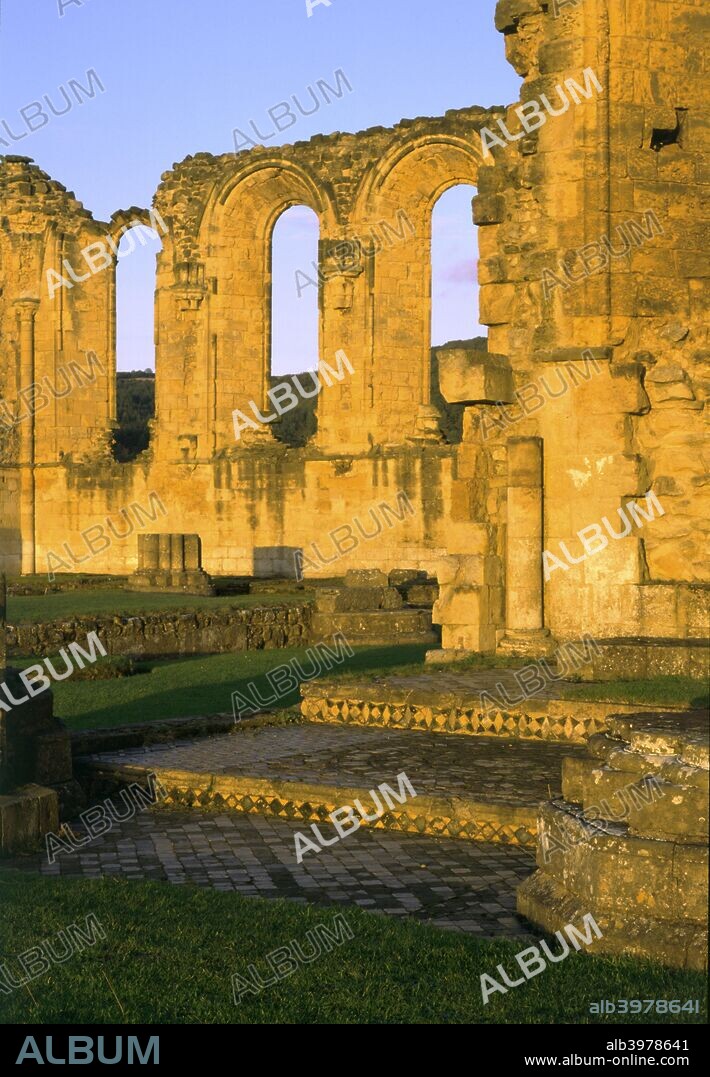The photograph showcases the facade of an ancient ruined building bathed in sunlight, casting a golden hue across its weathered bricks. The structure features prominent arched windows, though the roof is missing, and displays a timeworn, classic architectural style. At the bottom of the image, two steps leading up to the building can be seen, adorned with a distinctive darker design of squares or diamond shapes. Surrounding the building is uneven ground covered in patches of green grass. 

Across the photograph, the word "ALBUM" appears repeatedly in a light gray, almost off-white, all-caps text, diagonally positioned with varying degrees of brightness and translucency, creating a watermark effect. At the bottom of the image, a black strip displays the word "ALBUM" on both the lower left and right corners, along with the code ALB3978641 and the website www.albumonline.com. Above this strip, the same watermark is repeated, integrating both the ancient scene and the modern digital marking seamlessly. The sky above the ruin is clear blue, adding a tranquil backdrop to the historic remnants.